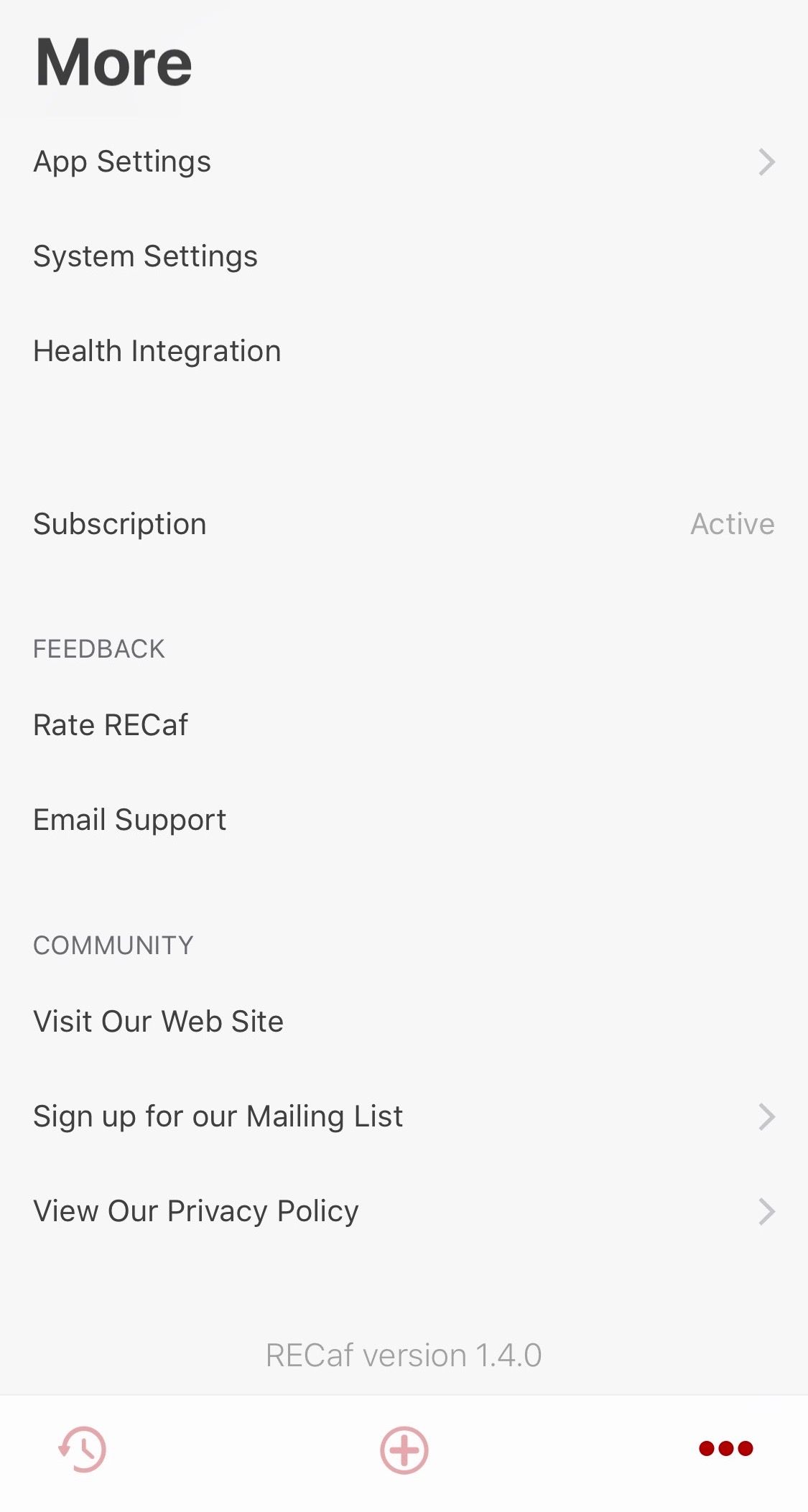This screenshot depicts the back-end settings interface of an application, primarily characterized by a gray background and black text. Prominently, at the top left, large black text labels the different settings available. The top section is captioned "App Settings," followed by "System Settings," "Health Integration," and "Subscription." To the right of these sections, the text indicates "Active" status.

Below this, there are two more sections: "Feedback" and "Community." The Feedback section includes options for "Rate Recap" and "Email Support." The Community section provides links to "Visit Our Website," "Sign up for our Mailing List," and "View our Privacy Policies," each accompanied by a forward arrow icon on the right side.

At the very bottom of the screen, the version of the application is displayed as "Recap Version 1.4.0." Also present are three circular icons: a refresh icon positioned on the left, a plus icon encircled in the middle, and three dots arranged vertically on the right, all in a distinct red color.